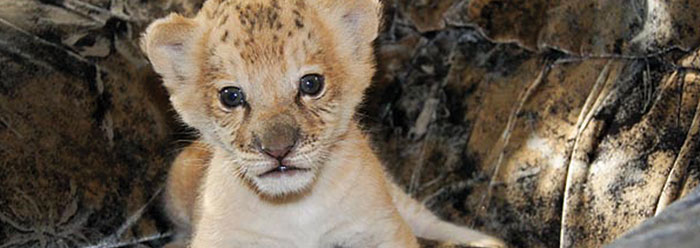The image depicts a very young big cat, possibly a lion cub, though there's some uncertainty due to its distinct markings. The cub has a mix of white to whitish fur in some areas, transitioning to tan and golden brown in others. Its forehead features noticeable black flecks or spots, and it has dark eyes that appear almost gray. The kitten has small, pointed ears, a black mouth, and a light pink nose. Despite the overall cuteness of the cub, it seems to exhibit a confused or startled expression. The background is dark and indistinct, possibly a tarp or blanket, but nothing specific can be determined about its surroundings, as the image is tightly cropped to focus on the cub.